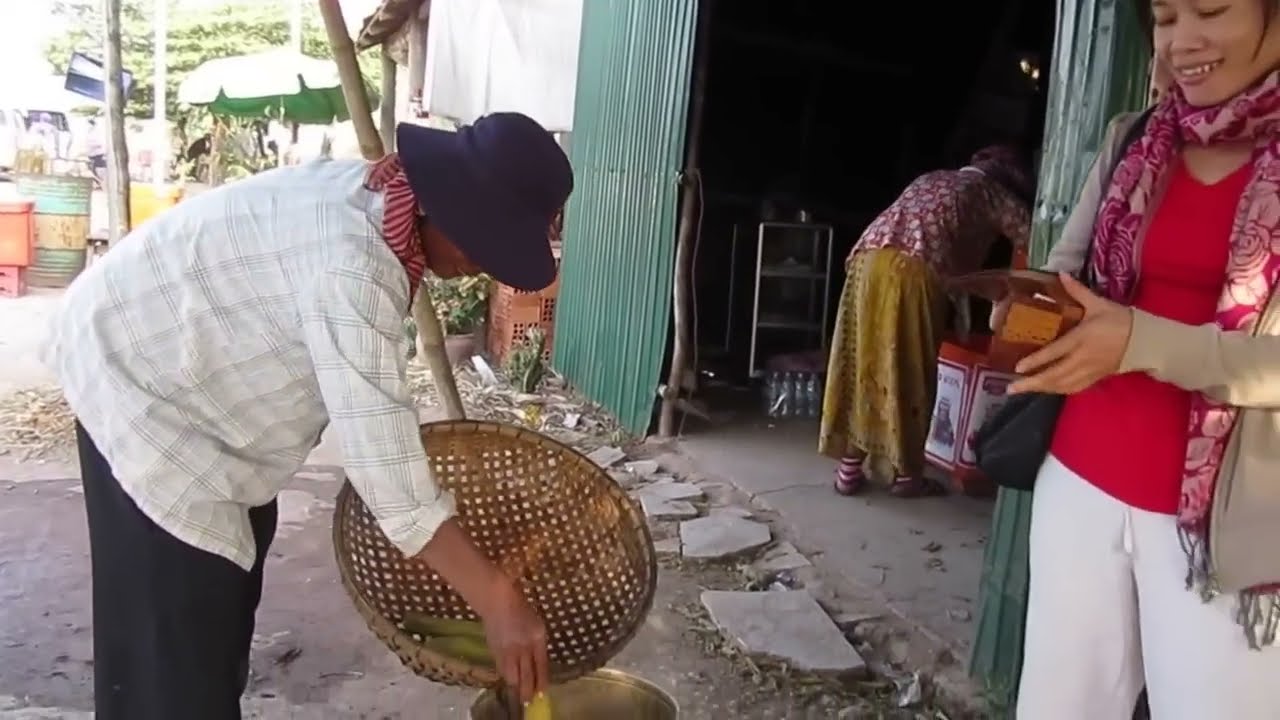In the image, three women are depicted in a bustling market scene, possibly in Southeast Asia. In the foreground, a woman clad in a black bucket hat, a red scarf, a white flannel-patterned shirt with rolled-up sleeves, and black pants is bent forward, focused on dropping items from a large woven bamboo basket into a silvery yellow bowl that appears to contain soup. Her facial features are visible as she concentrates on her task.

To her right, another woman wearing a red shirt, a patterned red and pink scarf, and white pants is smiling with her top teeth visible. Her eyes are mostly closed as she looks down at an open brown wallet, seemingly ready to pay. 

In the background, a third woman is hunched over, busy with some work at a table. She is dressed in a light brown long skirt, striped socks, and a purplish shirt with white spots. The setting includes green double doors that lead to a metal warehouse-like building with corrugated metal walls and sliding doors. This woman appears to be attending to a cart positioned inside this metallic structure. The overall ambiance of the scene is lively and industrious, evoking the essence of a local market.